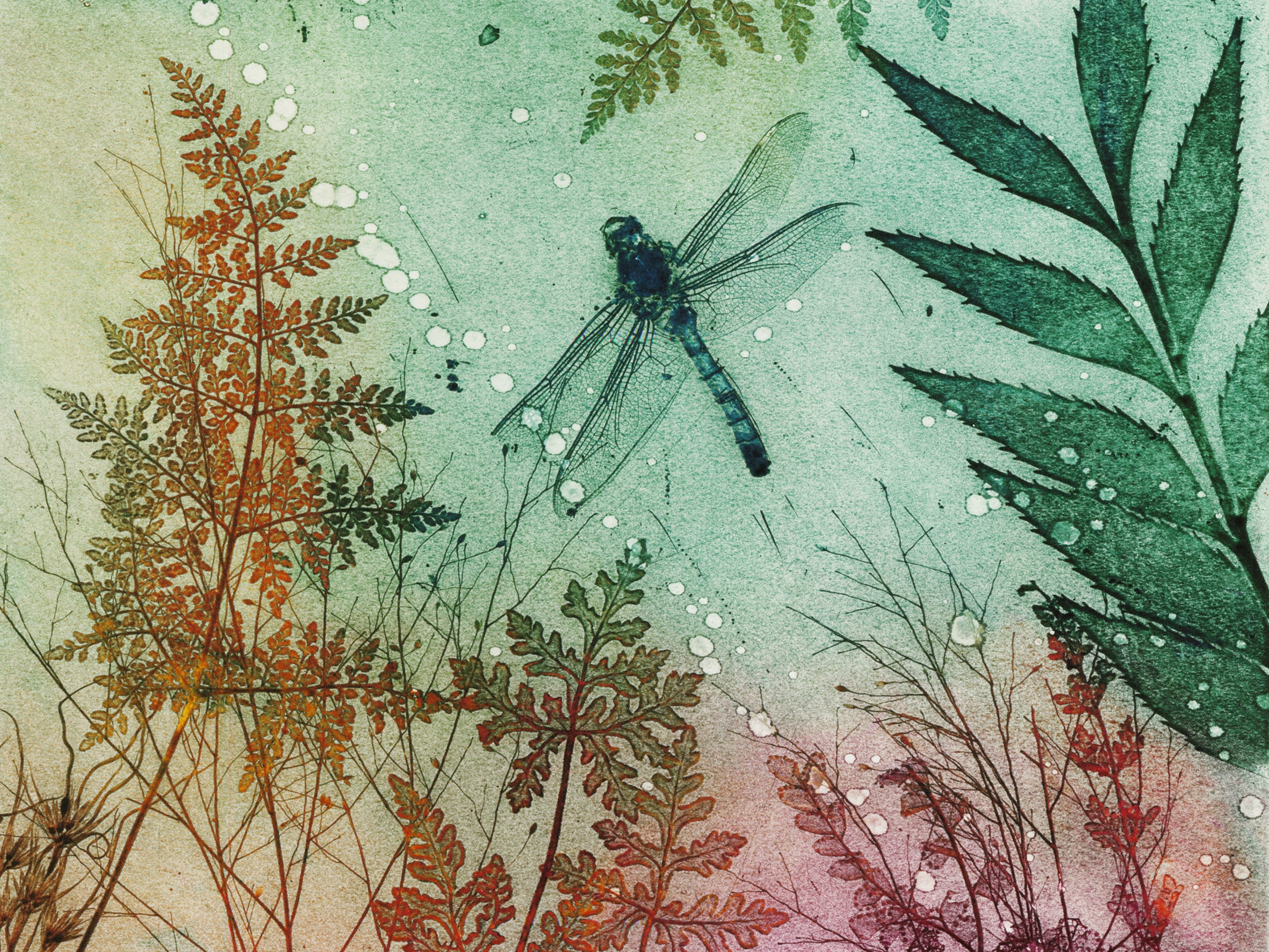This image portrays a vintage-style watercolor artwork with a soft pastel palette. Dominating the scene is a large dragonfly with aqua and greenish-black hues, positioned prominently in the middle of the painting. Its delicate wings span wide, tinted with subtle greens. The background features a blend of light aqua and maroon tones, elegantly faded by what appear to be water droplets or beads, creating the illusion of water spots across the surface. Surrounding the dragonfly are an array of leaves and ferns in various colors, including green, rust, crimson, yellow, orange, and pink. Ferns cascade from the top, rise from the bottom, and intermingle with different hued leaves, creating a rich, textured tapestry. The interplay of colors and droplets gives it an exquisite, ethereal quality, capturing the essence of nature in a delicately balanced composition.